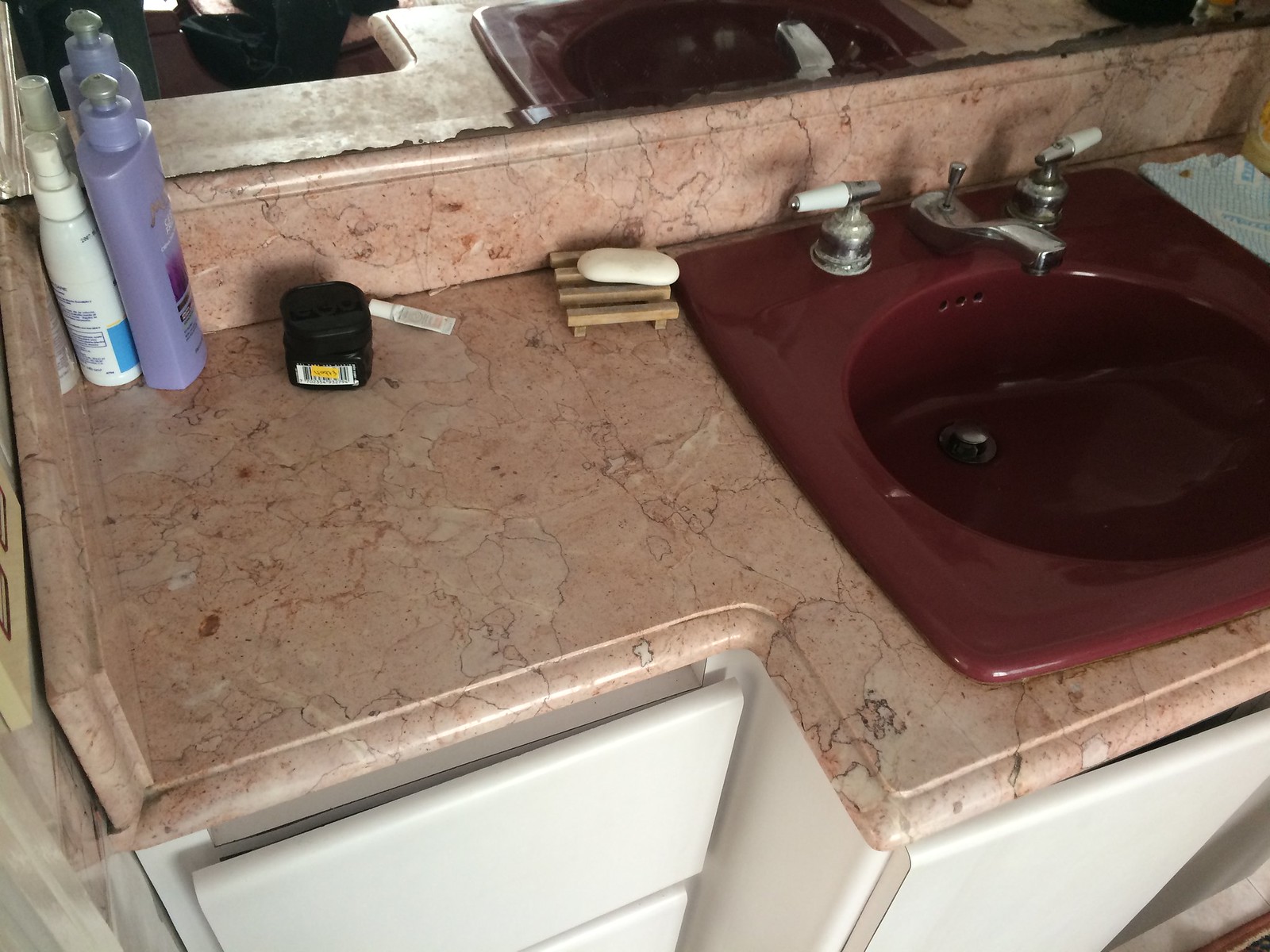This image showcases a home bathroom, focusing primarily on the countertop and sink area. The countertop appears to be made of marble with a pinkish or rose hue. Centered on the counter is a burgundy or maroon-colored sink, complemented by chrome faucets and handles that feature white accents. The faucet handles are distinctly separated, not mounted on a shared base.

On the left side of the counter, there is a variety of personal items: a spray bottle (possibly containing hairspray), another unidentified bottle, a black jar, a small white tube, and a wooden soap tray holding a bar of soap. To the right, a cloth, rag, or paper towel is seen alongside another bottle.

In the background, a mirror reflects parts of the bathroom, including a glimpse of the toilet. The vanity below the counter is equipped with white drawers and cabinet doors, offering storage space. The overall scene gives a sense of a well-used and personalized bathroom space in a residential setting.